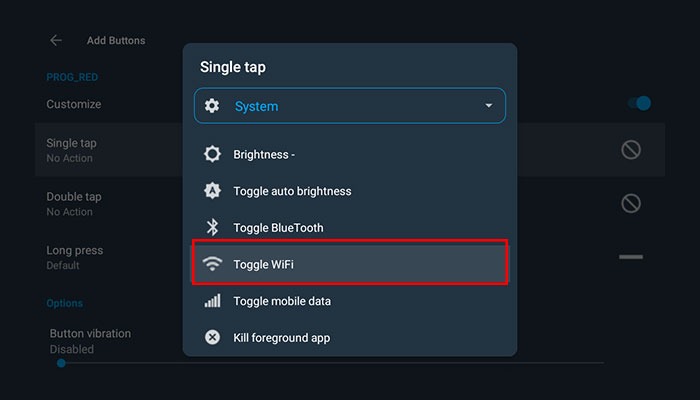The image is a screenshot of a settings page on a device, either a computer or a phone, which appears to be in dark mode. The main screen is dark, with several options grayed out due to an active dialog box taking the focus. Along the left side of the screen, partially obscured but still readable, there are setting options such as "add buttons," "customize," "single tap," "double tap," "long press," "options," and "button vibration."

Dominating the center of the screen is a dialog box specific to modifying single-tap gestures. The currently selected option in this dialog is "toggle Wi-Fi," highlighted by a red rectangular box surrounding the text. The drop-down menu at the top of the dialog reads "system," indicating that the user is making system-level changes. Below the drop-down menu, other selectable actions are listed, including "brightness," "toggle auto brightness," "toggle Bluetooth," "toggle mobile data," and "kill foreground app." The selection of "toggle Wi-Fi" suggests the user is configuring a single-tap gesture to control the Wi-Fi setting on their device.